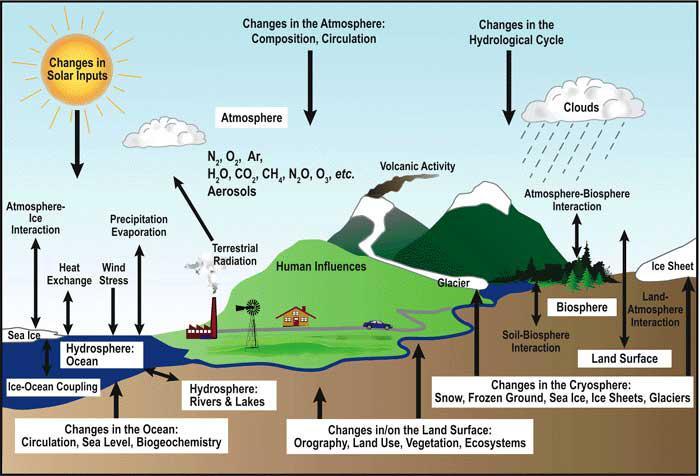This detailed digital illustration provides a comprehensive scientific diagram depicting the complex interactions within Earth's environment. It highlights multiple components and their reactions, including changes in solar input, atmospheric composition and circulation, and the hydrological cycle. The image prominently features a diverse landscape consisting of a high mountain, a volcano, green land, dirt patches, a lake, and a river. Numerous labels denote various environmental elements such as clouds, the Sun, sky, and wind stresses.

The diagram emphasizes interactions between different environmental elements like atmosphere-ice dynamics, ocean and air heat exchanges, and human influences, including activities like factory emissions and driving. It delves into the impacts on sea level, biochemistry, and terrestrial ecosystems. The roles of volcanic activity, terrestrial radiation, and aerosols are also illustrated. Additionally, the image covers changes on land surfaces, such as those involving glaciers, ice sheets, snow, and frozen ground, as well as ocean and ice coupling. Overall, it serves as a detailed representation of how various factors, including human activities, shape and influence the environment and Earth's biosphere.